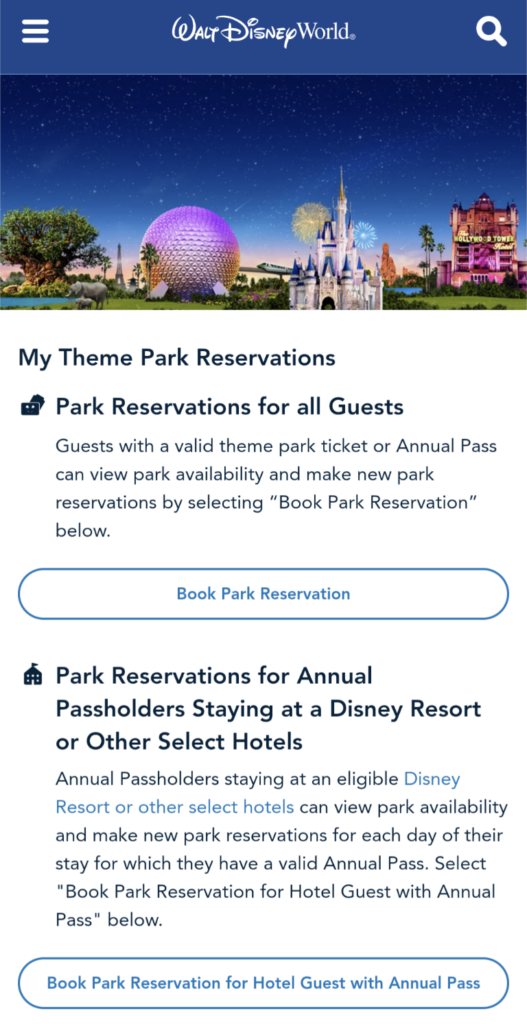This image is a screenshot taken from a mobile phone, displayed in a portrait orientation. At the top, a dark blue header spans horizontally across the screen, featuring a white hamburger menu icon on the left, cursive white text reading "Walt Disney World" in the center, and a white search magnifying glass icon on the right. Below this header is a vibrant composite image of Disney World, showcasing iconic landmarks from Magic Kingdom, Epcot, Animal Kingdom, and other parks set against a sky illuminated with fireworks.

Directly beneath the image, bold black text reads "My Theme Park Reservations." An icon and subsequent text below it state "Park Reservations for all guests," followed by detailed subtext explaining that guests with a valid theme park ticket or annual pass can view park availability and make new reservations by selecting the "Book Park Reservation" button below. This button appears as a long blue oval with white interior and blue text saying "Book Park Reservation."

Further down, an image of a building topped with a flag accompanies the text "Park Reservations for annual pass holders staying at a Disney Resort or other select hotels." Additional descriptive text follows, providing more information and concluding with another actionable button. This second button is also a long blue oval, with white inside and blue text indicating "Book Park Reservation for hotel guests with annual pass."